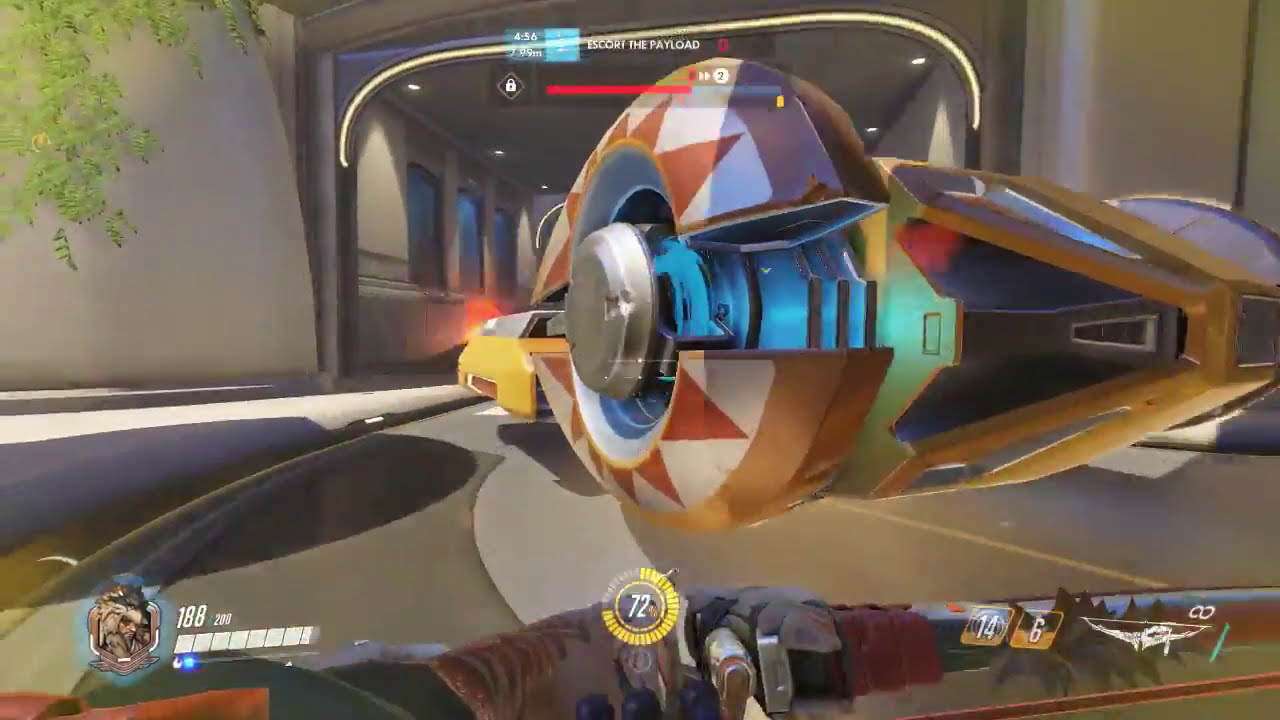The image is a detailed, color freeze-frame from a futuristic racing video game. Dominating the center is a vividly colored, futuristic flying vehicle characterized by its unique, vibrant design. The vehicle features a yellow and orange body with hints of red and blue reflecting off its sleek surface, accentuated by large hubcaps with a diamond-shaped pattern in rust and white, and glowing blue wheels. The vehicle appears to be flying down a hallway with blue windows in the background, suggesting a high-tech environment. At the top of the image, a progress bar with the objective "Escort the Payload" is visible, indicating the current task in the game. The bottom section of the image contains various navigational and game status details, including a speedometer and numerical indicators, such as '188' to the left, and '72,' '14,' and '6' in the lower right corner. There is also a smaller inset of the vehicle in a different scenario with additional navigational features. Adding more character to the scene, an evil-looking figure with white hair and possibly glasses can be seen on the left side, near a hanging plant, all set against a backdrop of a hallway with blue-lit windows.